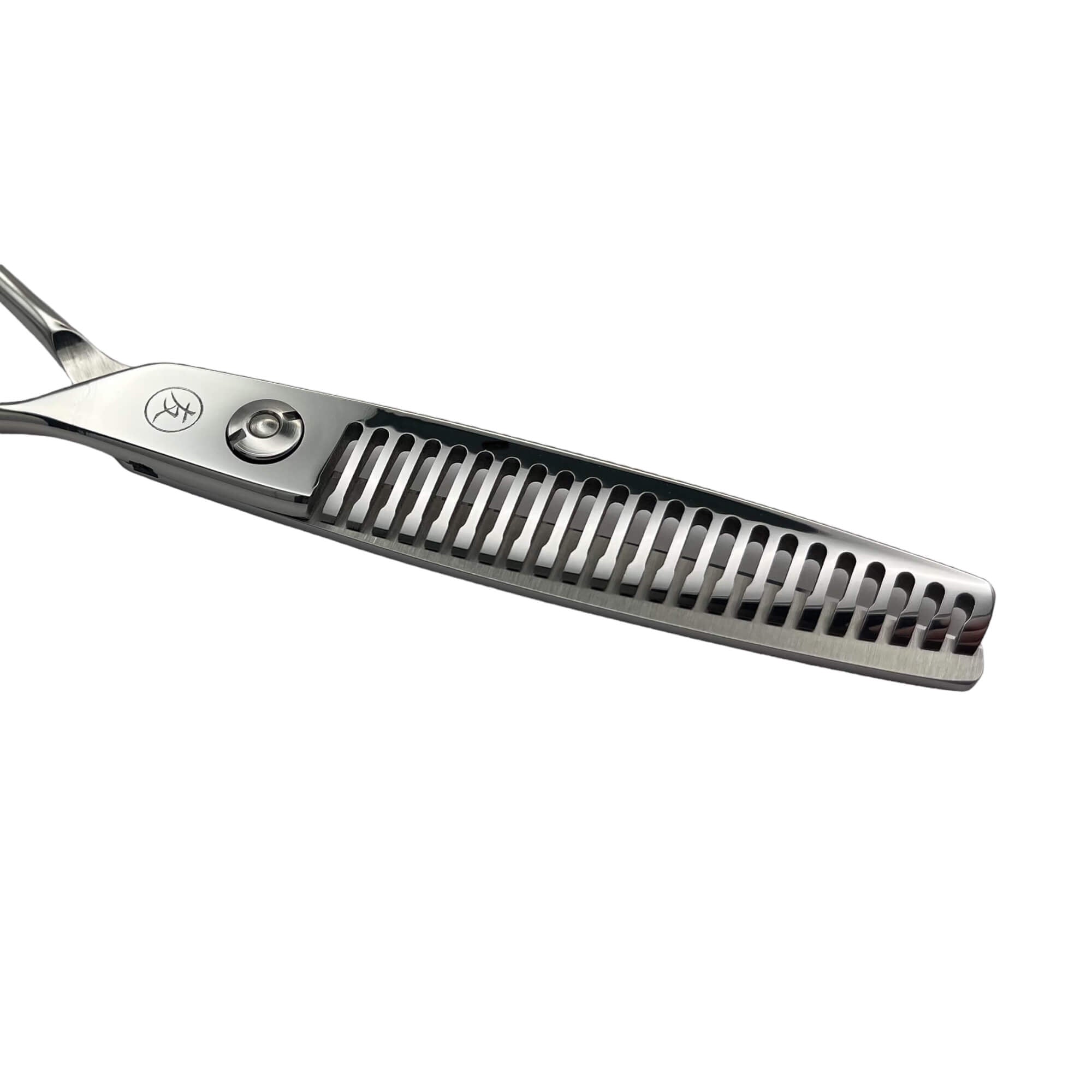The image depicts an assortment of metal clippings scattered across a pristine white background. On the left side, a prominent screw can be seen next to a mysterious symbol, which appears to be a Japanese or Asian character. Additionally, there is a pair of sleek scissors or a similar hair care tool placed near the left edge of the frame. The contrast between the cool metallic objects and the pure white backdrop underscores the intricate details of the scene.